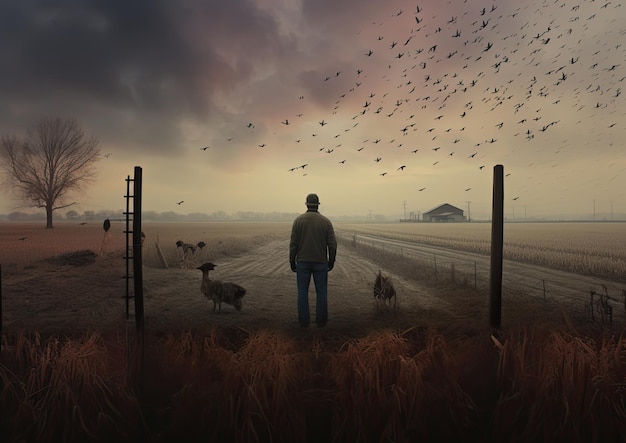In this evocative painting set in an autumnal farm landscape, a man wearing a backwards baseball cap, a jacket, and blue jeans stands in the middle of a dirt road bordered by fields of dried, brownish wheat or corn. Flanked by tall poles, he seems to survey his surroundings, which include a mix of animals, possibly goats or sheep, grazing and wandering around him. Surrounding the man are additional creatures, including birds and tumbleweed-like plants scattered across the ground. Dominating the sky, a large flock of birds flies overhead, mostly concentrated on the right side. The left side of the image features a leafless tree, and in the hazy background, a farmhouse or barn is visible. The sky, tinged with green and a hint of pink, adds an otherworldly atmosphere, enhancing the sense of solitude and reflection in this autumnal setting.